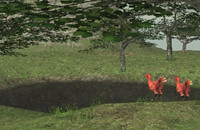A digital outdoor landscape image depicts a serene, verdant scene. Lush green grass extends across the foreground, leading to a variety of trees in the distance, each adorned with green foliage and slender gray trunks. Central to the image is a round pond with dark gray waters, which adds a tranquil element to the scenery. To the right of the pond, two birds stand side by side, both displaying vibrant orange plumage with distinct tail feathers and red heads, reminiscent of chickens or perhaps turkeys. The sky above is a soft whitish hue, suggesting daylight and enhancing the peaceful atmosphere of this natural setting.